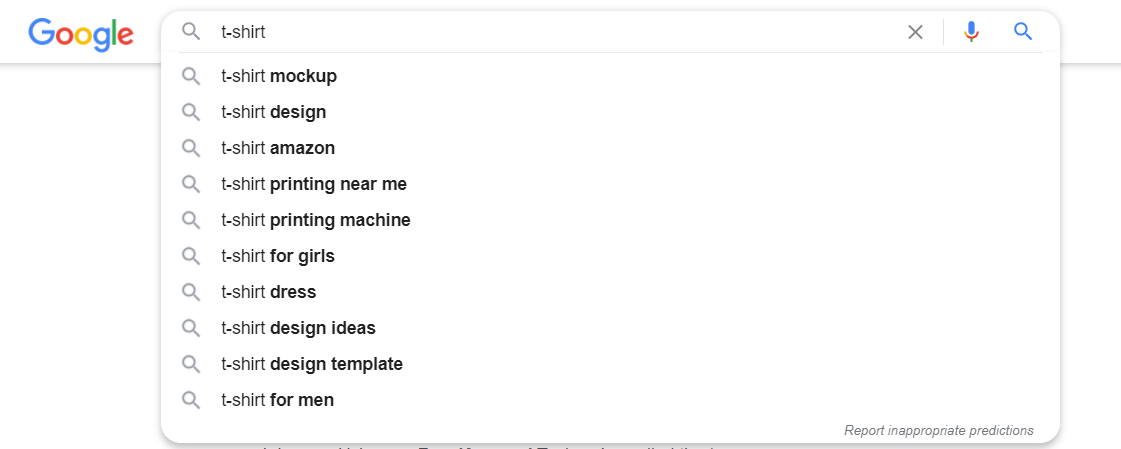This image is a screenshot from Google. At the top left corner, the word "Google" is prominently displayed in a sequence of blue, red, yellow, blue, green, and red letters. Centrally placed on the screen is a search bar with the queried term "t-shirt" appearing with a hyphen. Directly below the search bar are several suggested search results, including:

- t-shirt mock-up
- t-shirt design
- t-shirt Amazon
- t-shirt printing near me
- t-shirt printing machine
- t-shirt for girls
- t-shirt dress
- t-shirt design ideas
- t-shirt design template
- t-shirt for men

At the very bottom right corner, the phrase "Report inappropriate predictions" appears, providing an option for users to flag unsuitable suggestions. The image is entirely composed of text and lacks any photographic elements—a purely textual screenshot. There are no people, animals, birds, plants, flowers, trees, bridges, automobiles, helicopters, motorcycles, bicycles, or food depicted in this image.